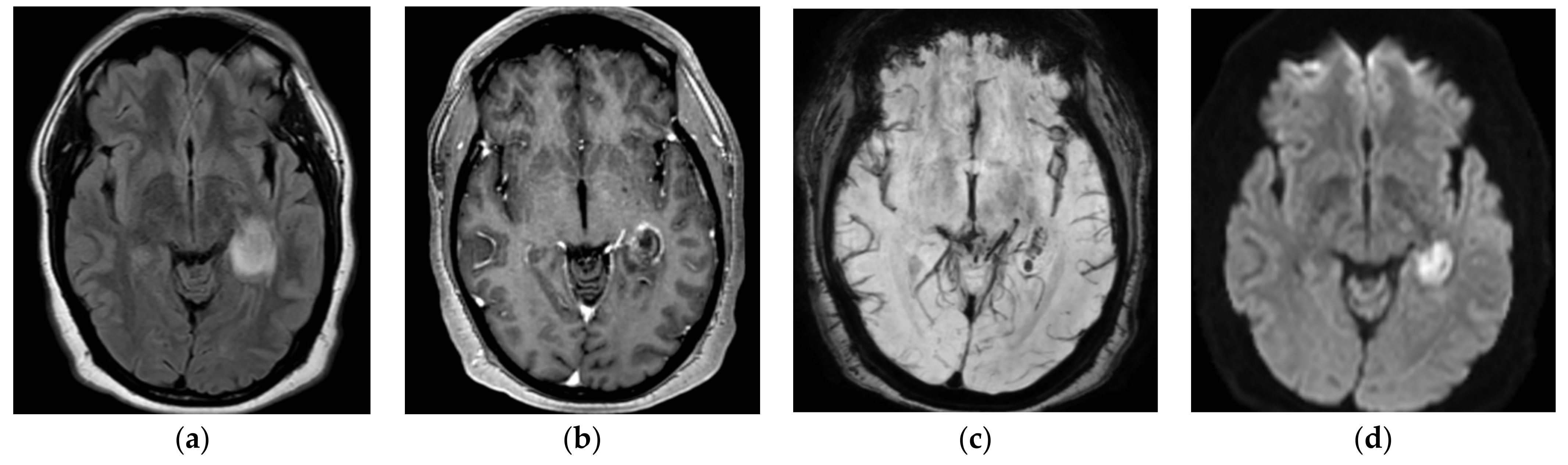This image is a detailed medical x-ray diagram of a human brain, provided by ABCMD, showcasing four different scans labeled A, B, C, and D. Each of these black-and-white images represents a cross-section of the brain from different perspectives and layers. Image A appears to be a top view highlighting the outer edge of the brain, enveloped by the skull. Image B reveals the texture and fluid areas surrounding the brain, indicating the brain's wetness. Image C provides a clear illustration of the brain's nerve structures, while Image D focuses solely on the brain tissue without the surrounding skull. These scans together offer a comprehensive look at various components and layers of the brain.